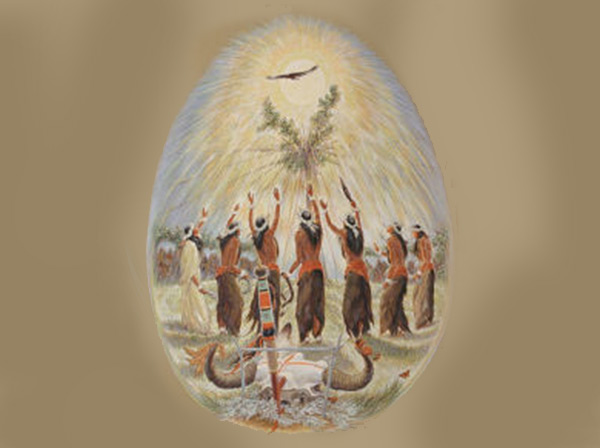The artwork features a central egg-shaped image set against a light brown, beige background. Enclosed within this shape are several Native American figures, possibly an indigenous tribe, characterized by their traditional attire that includes straw skirts with orange bands and white headbands, as well as long, dark hair. These figures are depicted with their hands raised, seemingly in worship or reverence, directed towards a prominent brown eagle soaring in a sunlit sky adorned with cascading rays. Below the eagle, a tree branch is visible. On the ground, lying amidst gray ashes from a fire that isn't burning, are various objects, including an animal horn and a spear with black, white, and orange stripes. The detailed representation captures a ritualistic scene filled with symbolic elements such as the eagle, the sun, and the raised hands of the worshippers.